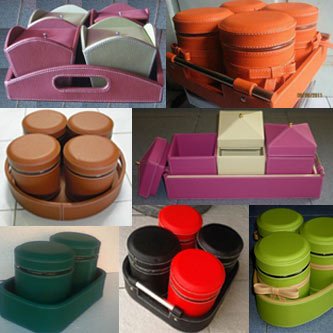This photograph is a product advertisement image displaying a grid of various containers, organized neatly to showcase multiple design options. The grid comprises rows with two or three images each, highlighting an array of colorful, organizational tools. In the top right corner, there are purple and white bins placed on a purple tray. Adjacent to this, in the top left corner, is a rose-colored tray filled with containers that resemble takeout Chinese food boxes, potentially made of painted wood or leather. Below this, there's a set of four small, round brown leather jars with lids. The grid continues further with an orange tray featuring orange jars, a green section containing two green containers, and additional black, red, pink, white, and orange containers, each placed on matching trays. This diverse collection illustrates the wide variety of storage options available to organize personal items.